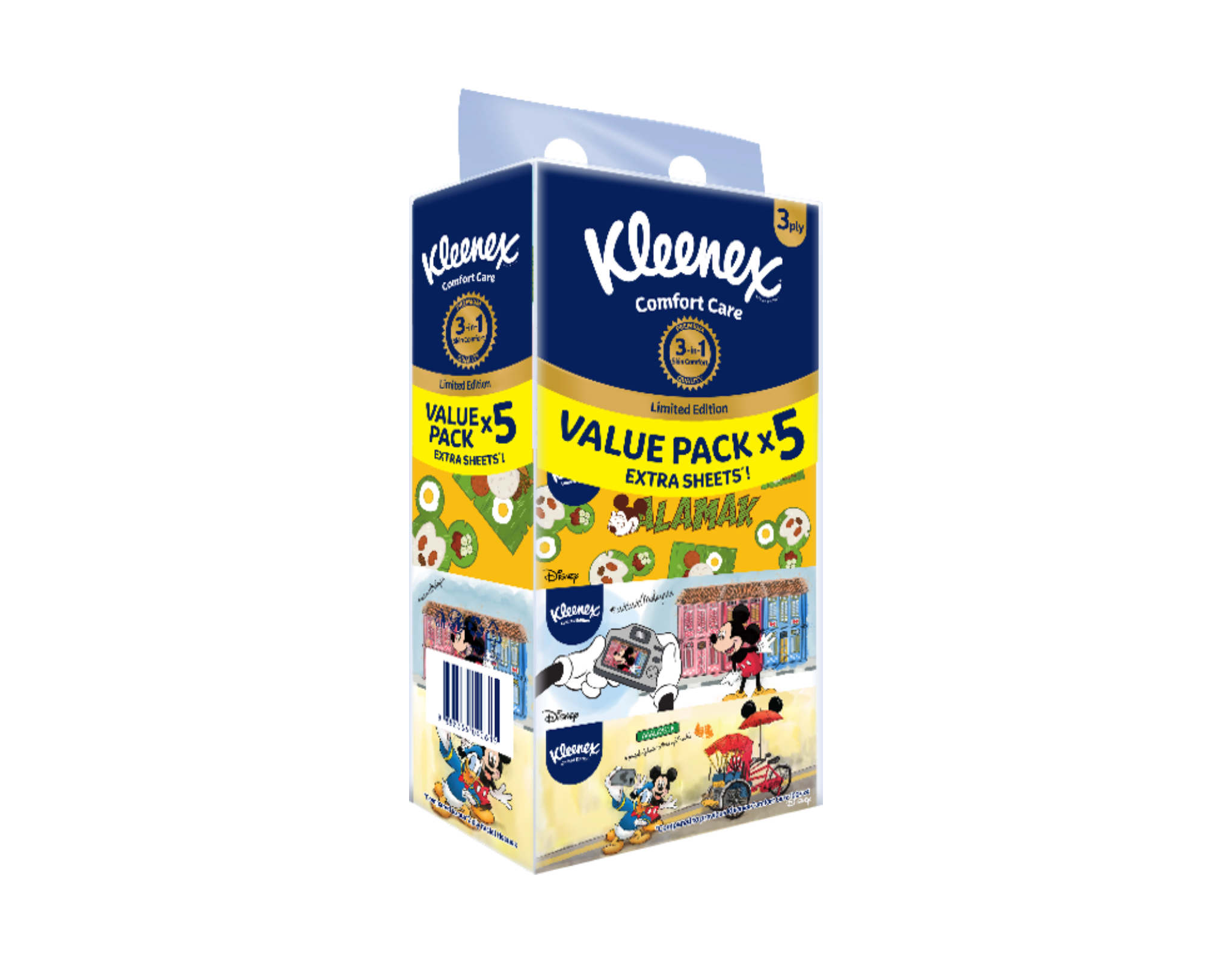The image depicts a Kleenex Comfort Care Limited Edition Value Pack of hand tissues. The packaging prominently features the Kleenex branding at the top in white text on a blue background. The box states that the tissues are three-ply and marketed as a '3-in-1' with five extra sheets, emphasizing its value with a 'Value Pack x 5' label. The design is Disney-themed, showcasing vibrant and colorful imagery of beloved characters like Mickey Mouse in various guises, Donald Duck, and Pluto. Scenes include Mickey Mouse hands holding a game controller, a souped-up tricycle with Mickey Mouse ears, and other playful Disney elements across the packaging. The background color transitions from dark blue to gold and then to bright yellow, each section aligned with specific textual information about the product. The image is presented as a cutout with a white background, angled partially to showcase both the front and side panels of the box.